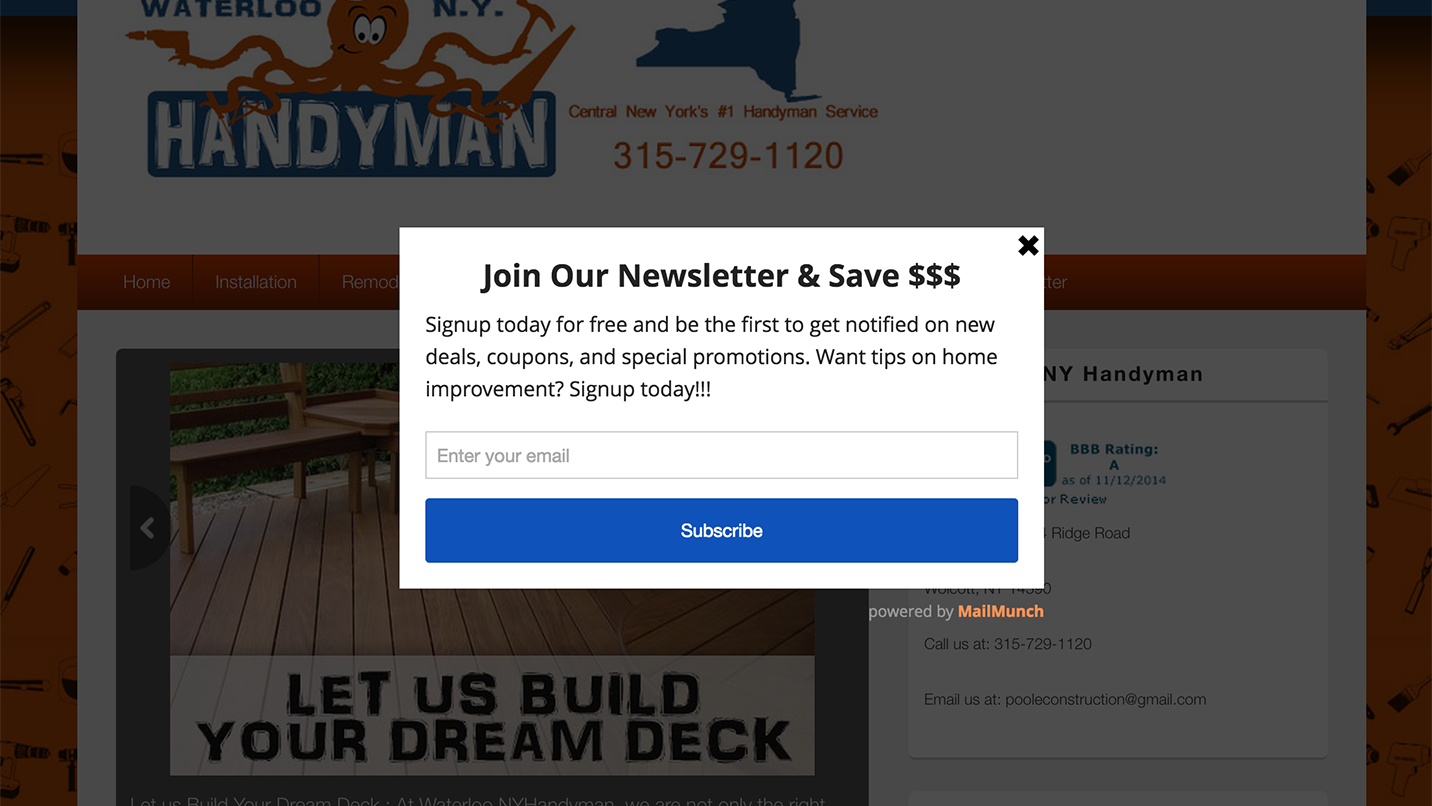The image is a screenshot of a website with a prominent pop-up blocking much of the view. Due to the pop-up, the background of the site has been overlaid with a very dark gray, opaque layer. Through this overlay, the website's primary background appears to be red, featuring white content boxes.

In the uppermost white box, a red octopus logo sits above a blue rectangle with the word "handyman" written in white bubble letters. To the right of this logo, there is contact information and a phone number. The subsequent section displays an image of a wooden deck complete with outdoor furniture, accompanied by the tagline "Let us build your dream deck." Adjacent to this section are additional details such as an address and more phone numbers, all partially obscured by the dark overlay.

The central pop-up box contains an "X" in the top right corner for closing it. The main text, bolded and center-aligned, reads "Join our newsletter and save $$$." Below this, in smaller print, the text encourages visitors to "Sign up today for free and be the first to get notified on new deals, coupons, and special promotions. Want tips on home improvement? Sign up today!!!" Following this enticing offer, there is a text box labeled "Enter your email," and a blue button below it with the word "Subscribe" in white. 

Overall, the screenshot captures a website offering handyman services, showcasing promotional content obscured by a pop-up invitation to join their mailing list for exclusive deals and tips.